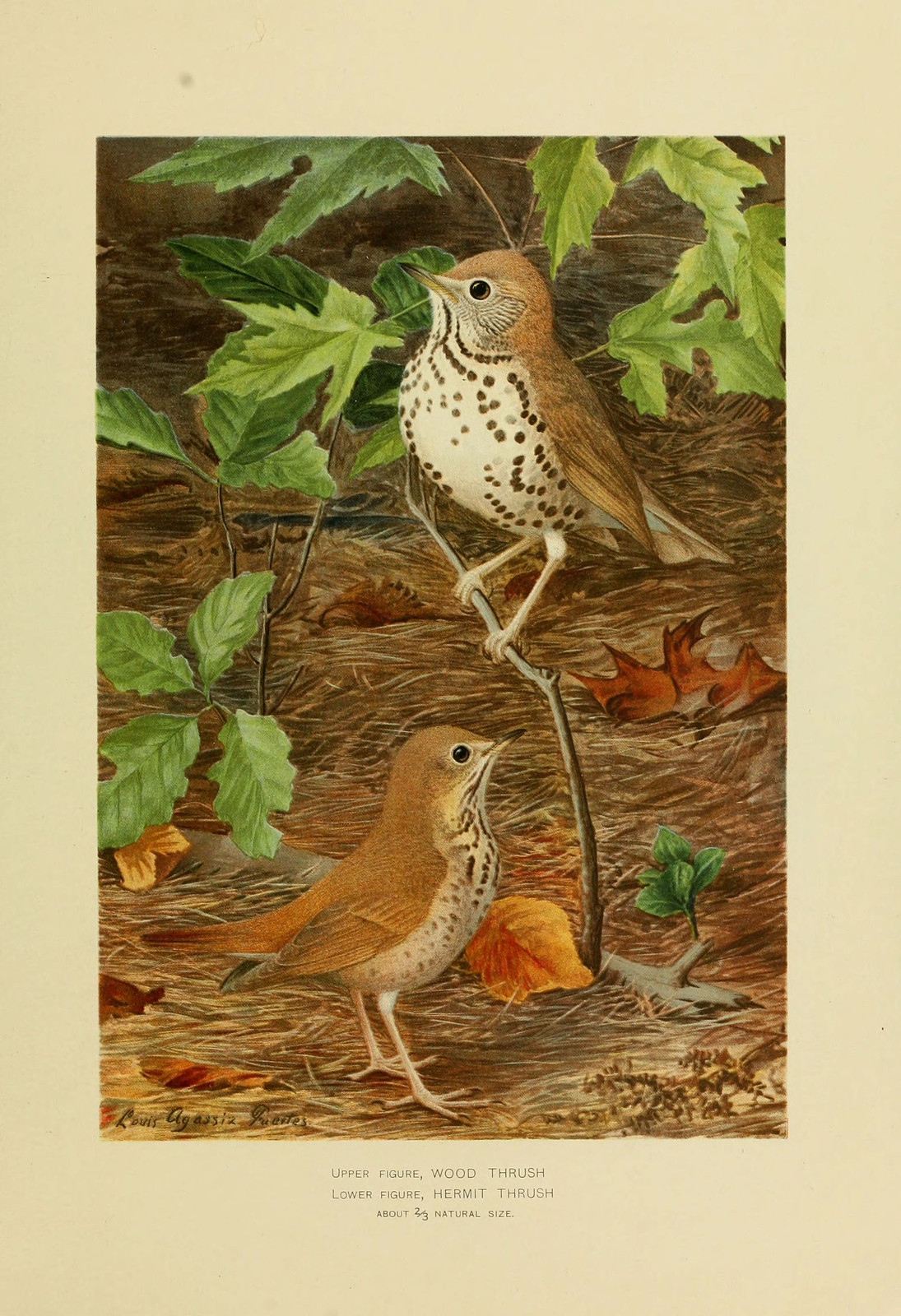This captivating painting captures two thrushes set against a natural landscape covered in twigs, grass, and an array of fallen and green leaves. One bird, identified as a wood thrush, is perched gracefully on a small twig protruding from the ground, its brown feathers complemented by black speckles on its chest and distinctive gray cheeks with a pointed beak. The other bird, known as a hermit thrush, is depicted walking along the ground with extended feet, mirroring the pattern of black dots on its brown-feathered body. Both birds are illustrated in different poses, with the wood thrush looking in one direction and the hermit thrush in another, adding a dynamic element to the composition. The background frame of the image is cream-colored, and in the lower left corner, the signature of the artist, Luis Agassiz-Priestiz, is visible. The bottom of the painting includes a caption stating "upper figure wood thrush, lower figure hermit thrush, about two-thirds natural size,” providing further context to the viewer.